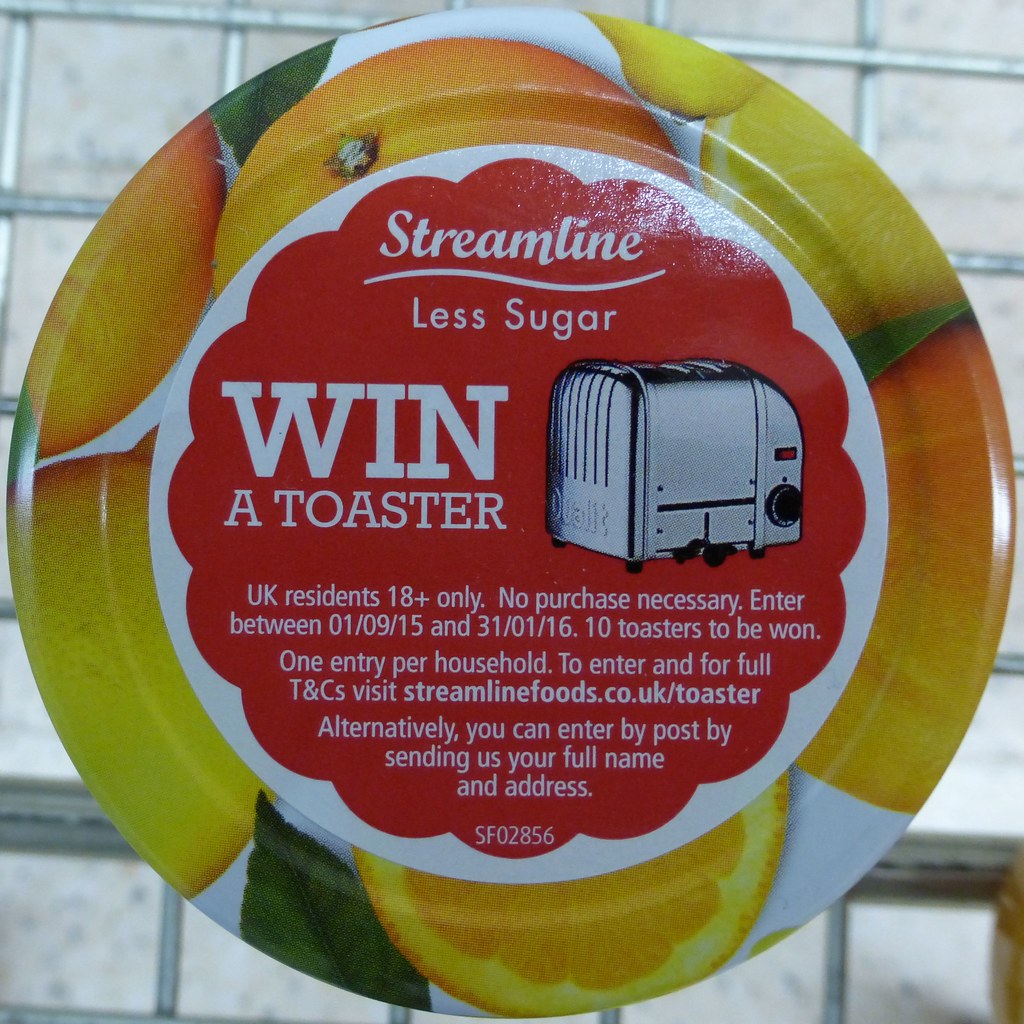The image depicts an advertisement that appears on a round, possibly metal, plate-like sign, which is the size of a typical plate and looks to be nailed to a tile wall. The border of the sign features images of oranges and leaves, creating a circular frame around the central content. Inside the plate’s white border, the background is red with a flower-like shape. At the top, the word "Streamline" is prominently displayed in large white letters, with "less sugar" written beneath it. The advertisement announces a contest with the bold statement, "Win a Toaster." On the left side of the image, there are details about the entry requirements, stating, "UK residents 18+ only, no purchase necessary, enter between 01/09/15 and 31/01/16, 10 toasters to be won, one entry per household." Additional text informs potential entrants to visit streamlinefoods.co.uk/toaster for full terms and conditions or to enter by post by sending their full name and address. On the right side of the ad, there is a shiny silver toaster image emphasizing the prize. At the bottom, a reference code "SF 02856" is noted.